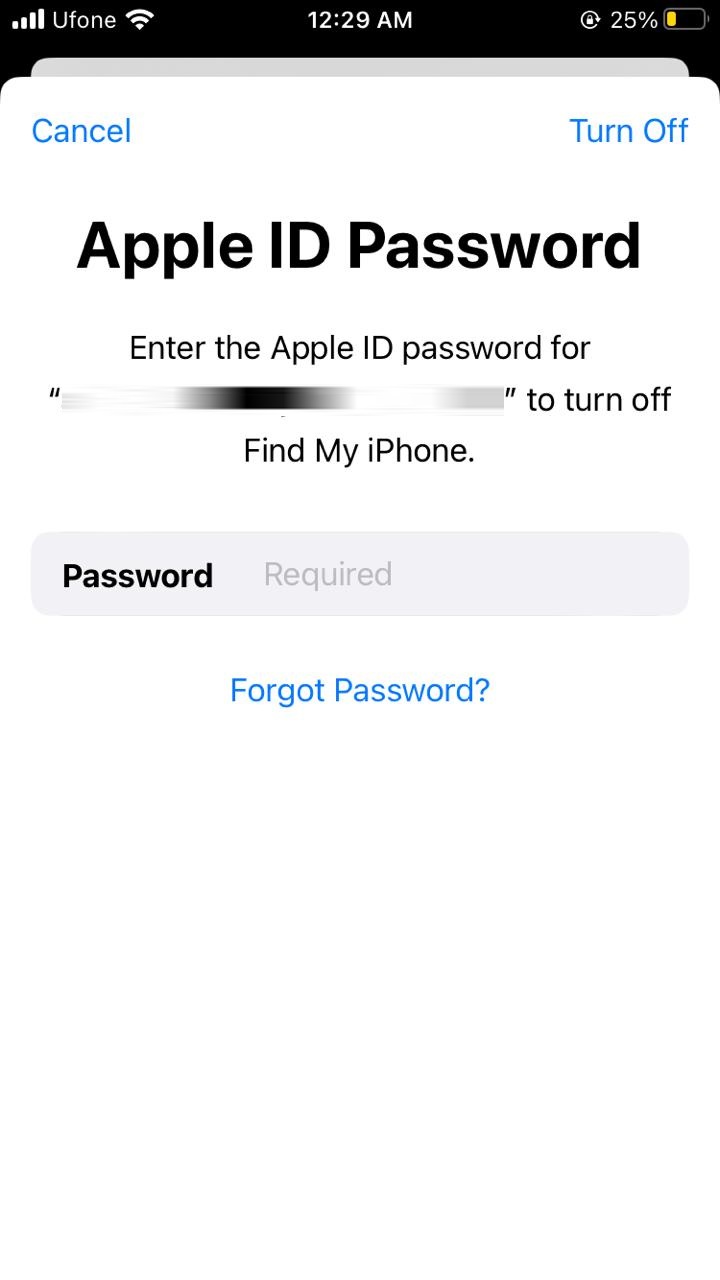A detailed image description:

This is a screenshot of an iPhone display featuring an Apple ID password prompt. The status icons at the top of the screen are highlighted: the battery life icon shows 25% remaining, indicated by a yellow battery bar. The screen rotation lock is active, ensuring the display does not rotate when the device is turned. The current time, displayed in white font, is 12:29 AM. Cellular reception is strong with four full bars, and the Wi-Fi connection is at maximum signal strength.

Centered below the status bar is a pop-up window titled "Apple ID Password." The top-left corner of this window features a "Cancel" option, while the top-right corner shows "Turn Off." The prompt requests the user to enter their Apple ID password and includes partially redacted text saying: "Enter the Apple ID password for [REDACTED] to turn off on my iPhone." Each text element within the screenshot is displayed in white font. The device model is identified as a "U phone."